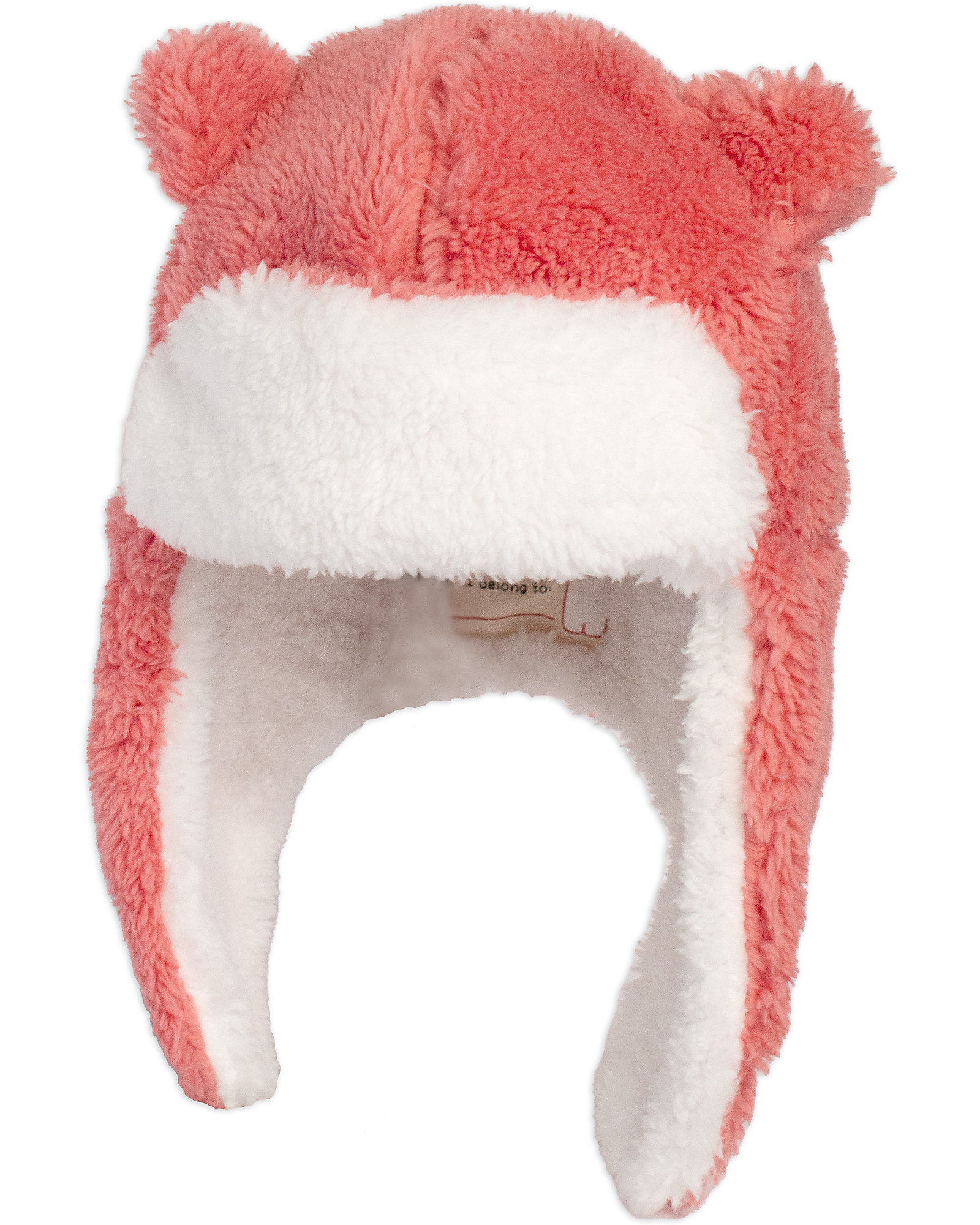This photograph showcases a whimsical novelty bear hat, primarily covered in a fuzzy, pinkish-orange fur with red hues. The hat features small, fluffy bear ears on either side, adding to its playful and childlike design. The interior of the hat, including the forehead area, is lined with plush white fur, creating a soft contrast with the outer color. A partially obscured label inside the hat indicates it is meant for a child, with a space to write the owner's name. The hat extends downward, forming flaps that cover the ears, cheeks, and neck, further enhancing its cozy and adorable appearance.